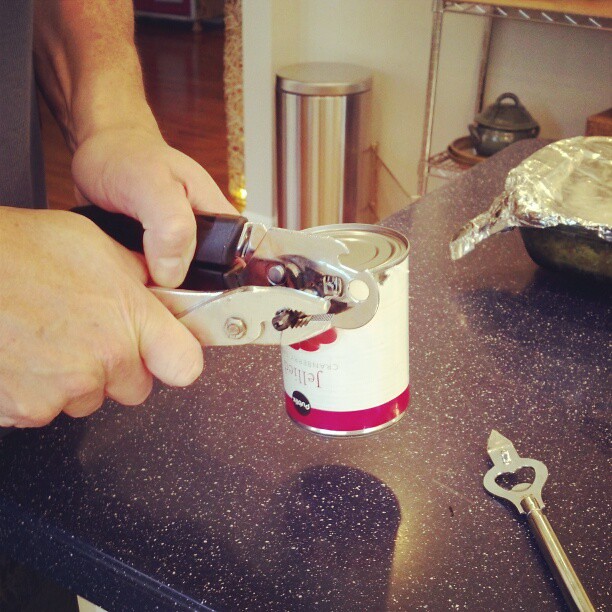In this square photograph, a Caucasian man, identifiable by the glimpse of his gray shirt, is opening a can of jellied cranberries, which is labeled upside down with pink text and a red stripe at the bottom, likely from the store Publix. The can hovers above a highly reflective black countertop speckled with white. The man is using a can opener and a wrench-like tool with both hands, which are visible from the left side of the image. To the right of the can, there is a metal object resembling a bottle opener with a sharp end, also placed on the counter. In the background, a covered casserole dish sits on the speckled counter. The setting includes a white wall in the rear, next to which stands a stainless steel garbage can and a stainless steel shelf laden with more kitchen utensils. A section of a hard wooden floor is visible to the left of the wall, completing the detailed and busy kitchen scene.